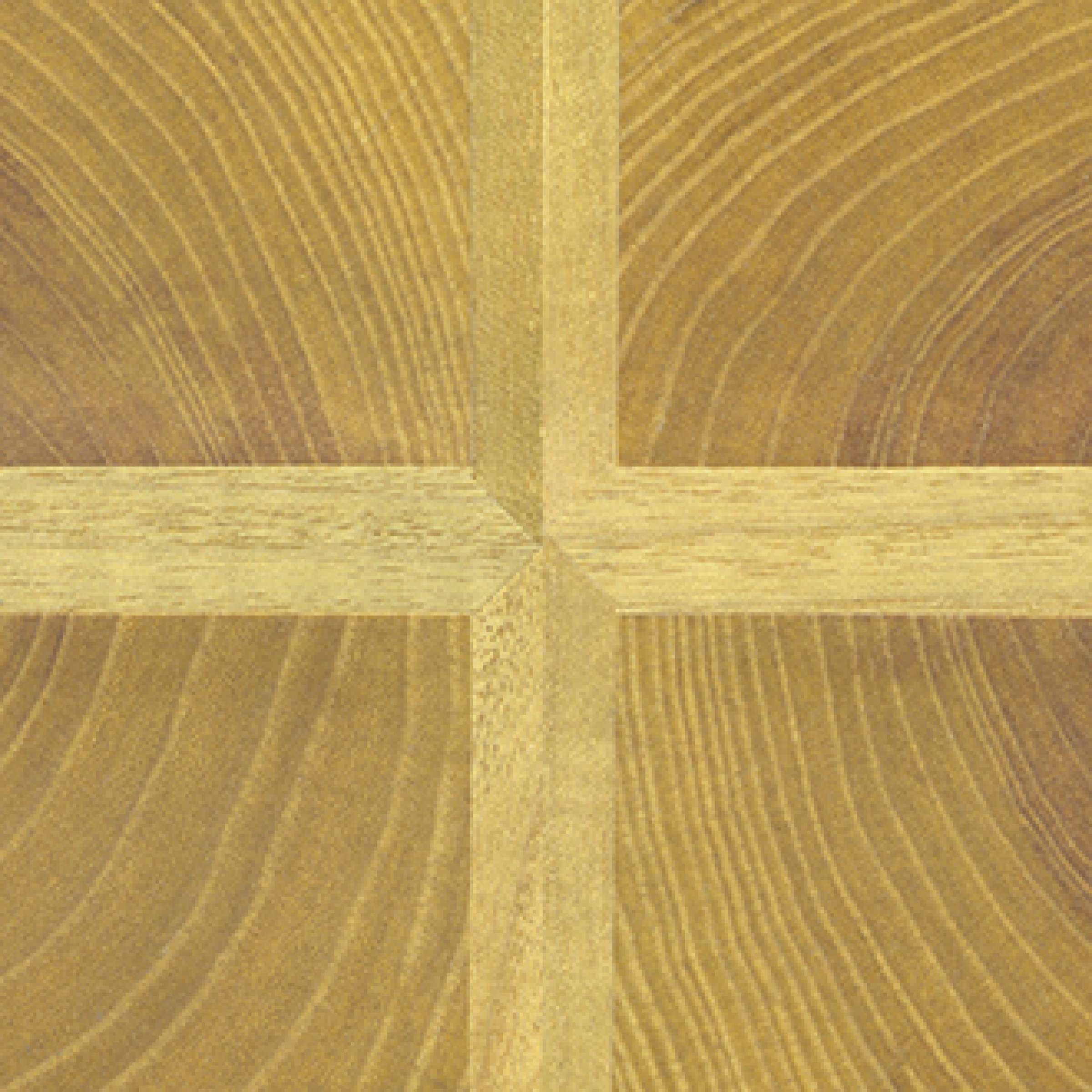This image depicts the top view of a square wooden table featuring a distinctive and intricate design. The table’s surface showcases a striking combination of wood grain patterns and angular divisions, creating a visually appealing centerpiece. The primary design consists of a cross pattern made from light tan wood that divides the table into four equal squares. Each of these sections is adorned with concentric circles, resembling the natural rings found in the cross-section of a tree, hinting at the table's organic origin.

The left and right halves of the table exhibit unique characteristics. On the left side, the circular grooves are spaced slightly wider, whereas the right side contains a larger, darker circle with tighter grain spacing. This contrast gives an impression of the wood being either from different sections of the same tree or from two separate trees, meticulously joined together.

The prominent cross pattern, approximately 2 to 2.5 inches wide, intersects at the center, creating a visually compelling X-shaped focal point. The harmonious blend of varied shades of darker wood within the four sections enhances the table’s aesthetic appeal, making it a remarkable piece of craftsmanship.